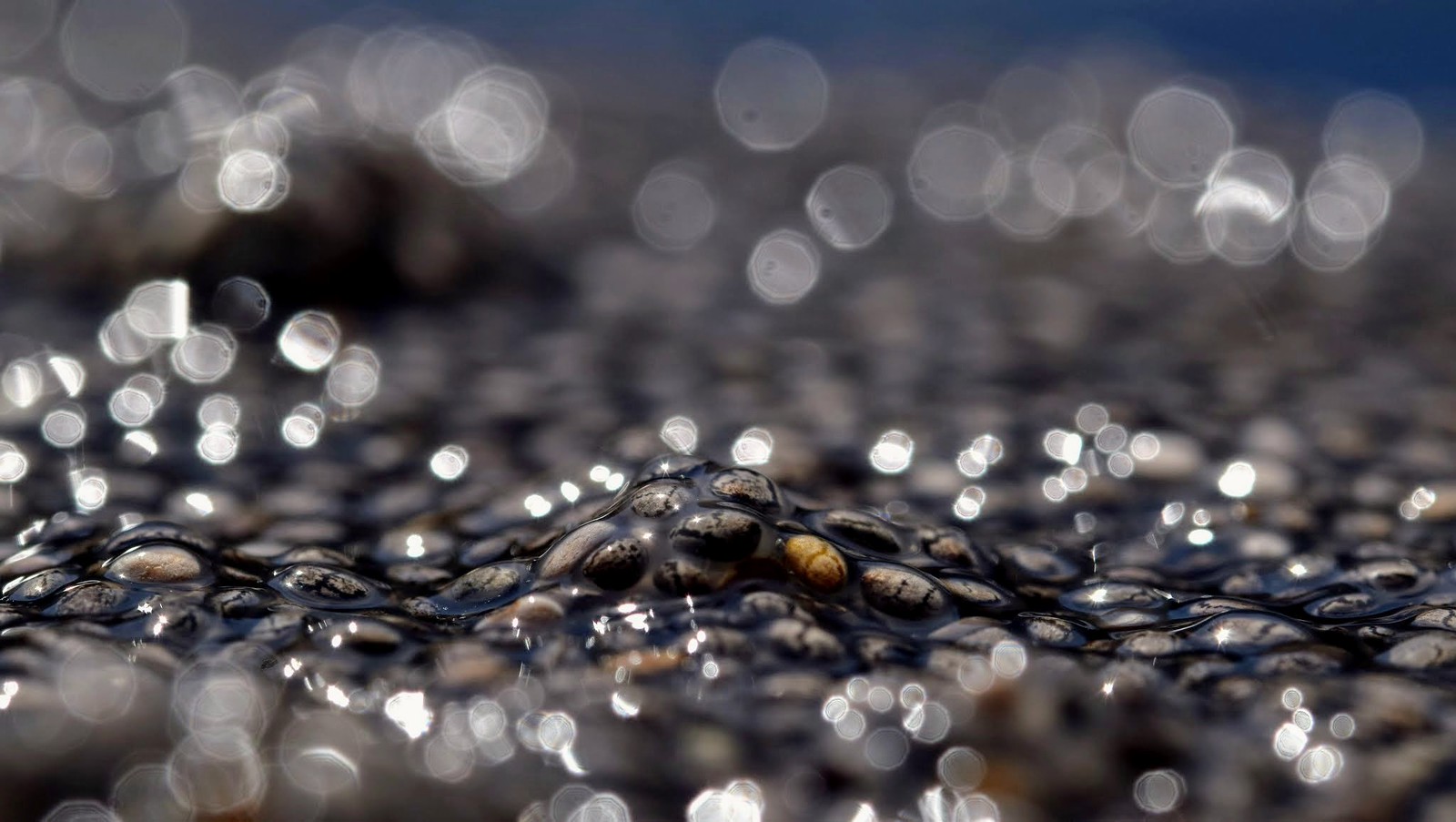This is a detailed and horizontally aligned rectangular photograph featuring a central in-focus area surrounded by blurry sections. The top part of the image is dark blue, reminiscent of sky, and is dotted with faded gray and white circular spots, which resemble water spots or reflections. These spots are denser on the left middle portion. The focused central area, running horizontally, showcases a formation of pebbles or rocks. These pebbles vary in color, including gray, brown, orange, and gray with black spots, forming a wavy, undulating pattern with slight inclines and declines, suggesting the appearance of tiny hills or slopes. Interspersed among the colorful pebbles are sections of black rocks, sometimes appearing to form a mound or unique pile. Water appears to trickle through this arrangement, creating reflections that glimmer like sunlight. The bottom portion of the image returns to a blurred area with similar water spot patterns. The entire scene projects a unique texture and the interplay of light on the rocks and water gives it an almost glittering effect, making it appear almost surreal and artistic.